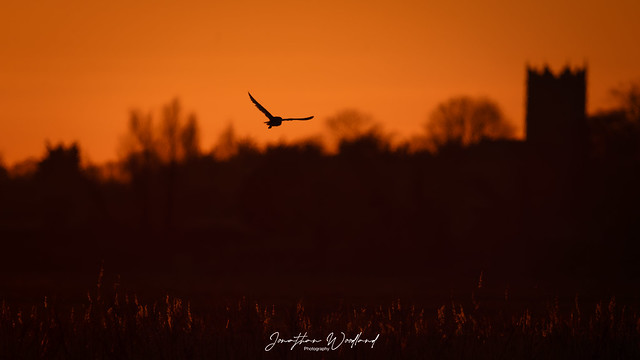This captivating photograph by Jonathan Woodland, entitled "Jonathan Woodland Photography," features a bird of prey, possibly a hawk, soaring gracefully through the sky. The image, taken during either sunrise or sunset, showcases a striking dichromatic palette of black and orange. The sky is bathed in a deep orange hue, suggestive of the golden hours of dawn or dusk. The bird, positioned slightly left of center, is sharply focused, highlighting intricate details of its feathers and wings in mid-flight. Below the bird, the field is barely visible, with faint, illuminated flecks of grass or grain at the bottom. The blurred background reveals outlines of trees and a hint of a distant building, adding an air of mystery. Centered at the bottom of the image is the photographer's signature in white cursive, further emphasizing the artistic composition and eerie, yet tranquil, atmosphere of this monochrome masterpiece.